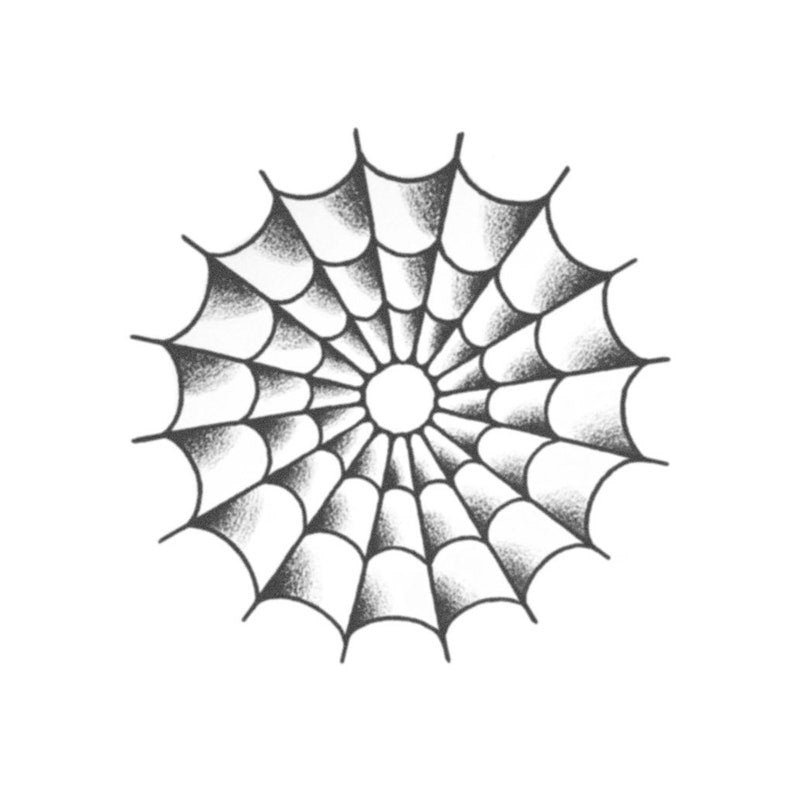The image is a detailed drawing of a spiderweb design, meticulously illustrated in a grayscale palette with precise black and white shading. The spiderweb has three concentric circular layers, each successively smaller towards the center, culminating in a hole at its core. The areas between the web strands are shaded in a gradient style, moving from dark to light, which gives a three-dimensional effect. The shading appears to have been done with a black colored pencil or a similar tool, adding a grainy texture reminiscent of an old-time comic or a precise computer-generated sketch. The design is perfectly symmetrical, and the entire composition is set against a plain white background, enhancing its intricate details.